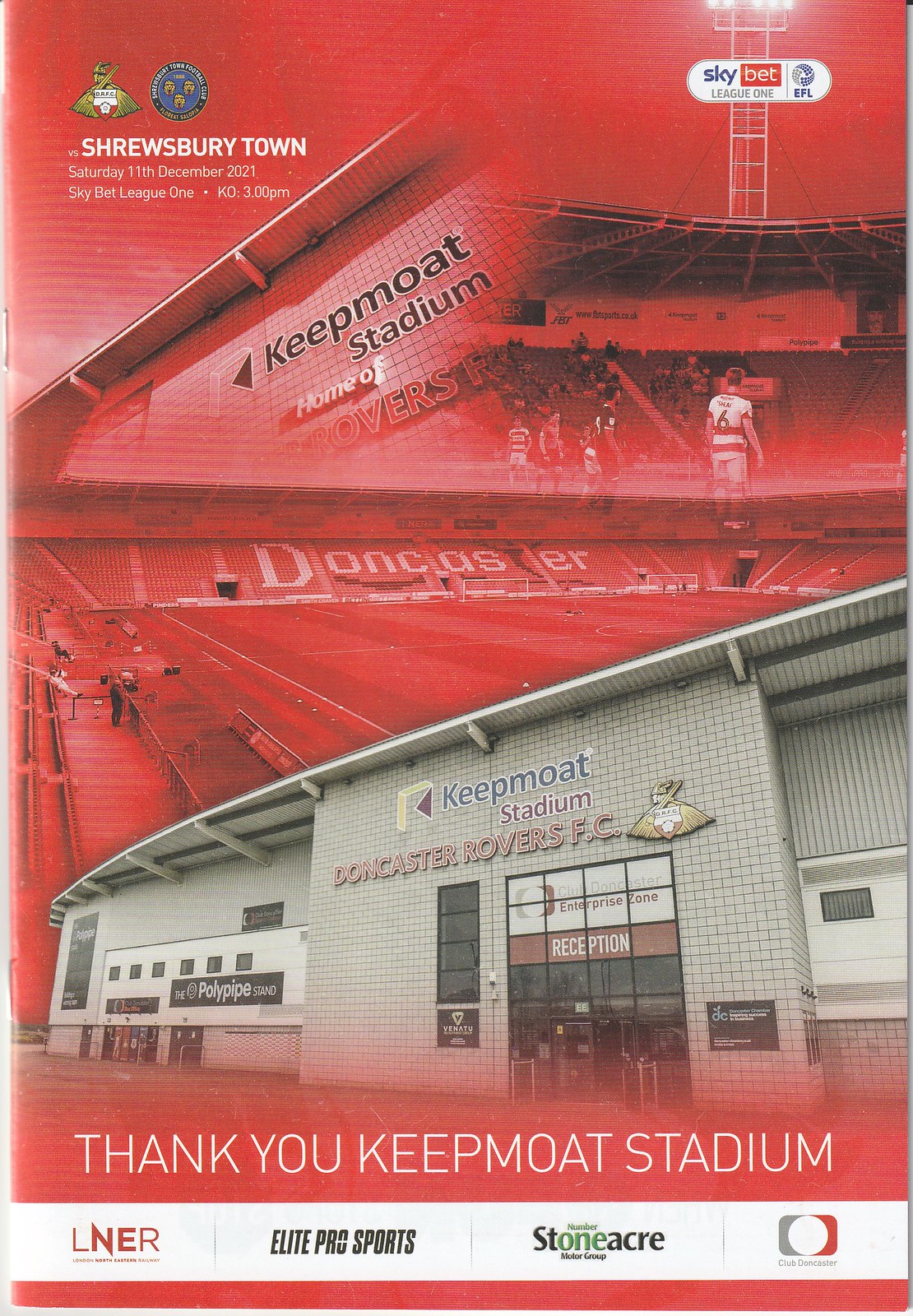The image is a promotional poster for the Keepmoat Stadium with a predominantly red background, accented with white and gray elements. At the very top, it lists the event details: "Shrewsbury Town, Saturday, 11th December 2021, Sky Bet League 1, 3 p.m." The upper right corner features the Sky Bet League GFL logo, while the top left corner includes various football team logos. Central to the image is a sign reading "Keepmoat Stadium" in red and blue letters, alongside "Doncaster Rovers FC". The bottom of the image showcases an entrance to the stadium with white brick walls and visible doors. Below this, there's text in white stating, "Thank You Keepmoat Stadium." Sponsors listed at the bottom include LNER, Elite Pro Sports, Stoneacre, and an indistinct logo resembling the NFL's emblem. Additionally, the background faintly depicts a football field with "Doncaster" visible in the stands, and players can be seen in the distance.